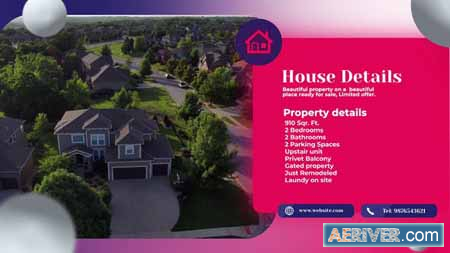The image displays a vibrant and detailed aerial view taken from a desktop computer screen, showcasing a large house amid lush greenery. The central focus is the expansive house, featuring a gray roof, white-trimmed windows, and walls. Noteworthy elements at the front of the house include what appear to be two garage doors. This house is surrounded by a rich tapestry of green grass and dense trees, reflecting a serene suburban setting. In the background, rooftops of additional houses are visible, nestled within the verdant landscape.

On the right side of the image, text on a red background reads “House Details” in white font, accompanied by smaller, unreadable text below. Further down, the text “Property Details” is also visible in white. The upper portion of the image features a soft pastel pink and grayish-purple background, enhancing the image’s colorful detail. In the lower right corner, a blue rectangular frame displays the website "ariver.com".